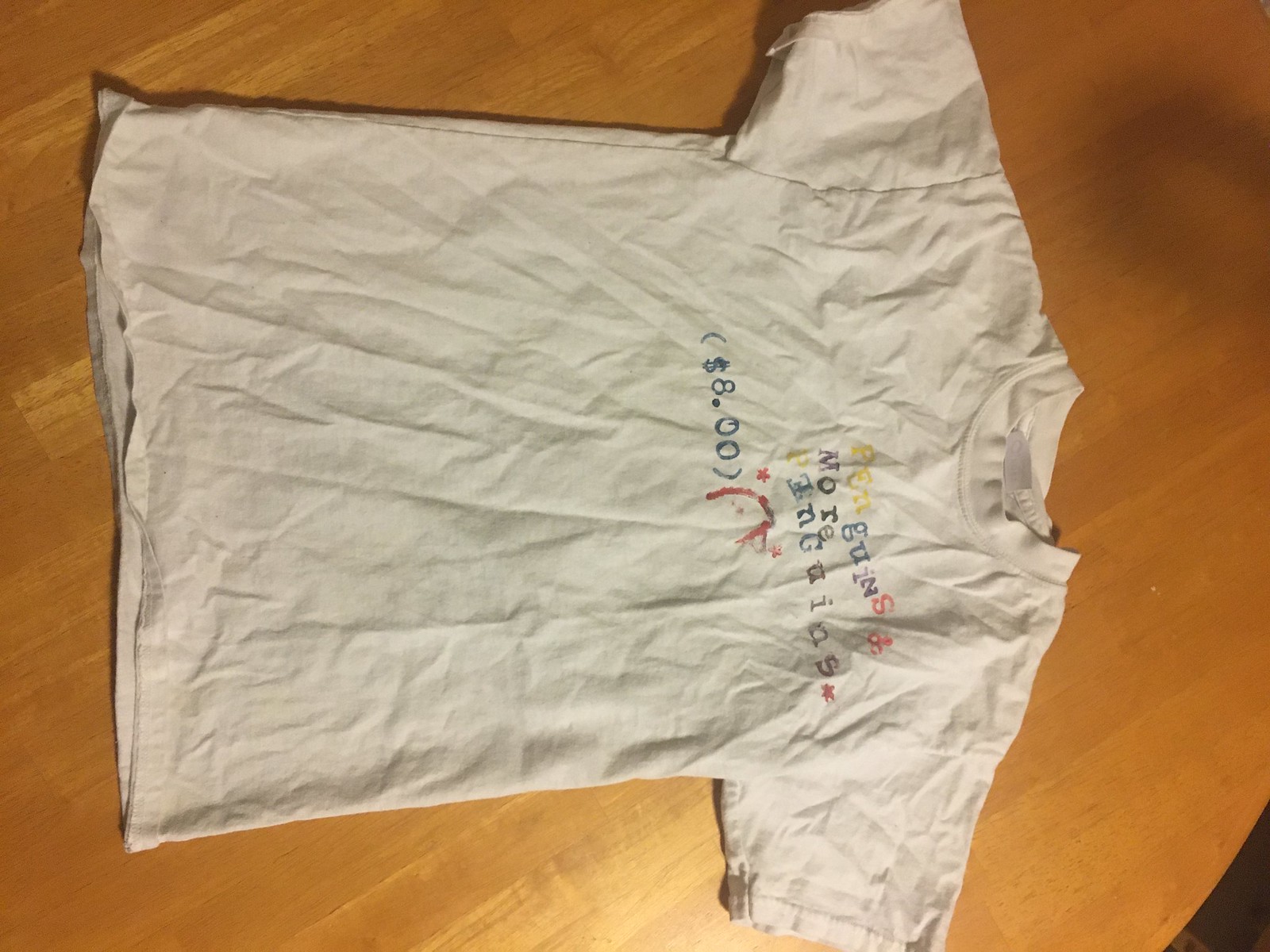This is a detailed photograph of a child's short-sleeved white t-shirt, lying sideways and flattened out on a light wood-colored, rounded table. The table has a dark background visible in the lower right corner. The t-shirt features a thick white crew neck collar and is heavily wrinkled. Across the chest area, there is multicolored writing in yellow, blue, red, purple, and gray letters that resemble a ransom note, spelling "Something guns more penguins" in a chaotic and slanted manner. There is also a crude red cartoon figure of a bird, possibly a penguin or chicken, evident by its beak. In the center of the shirt, printed in blue font within parentheses, is the price "$8.00."